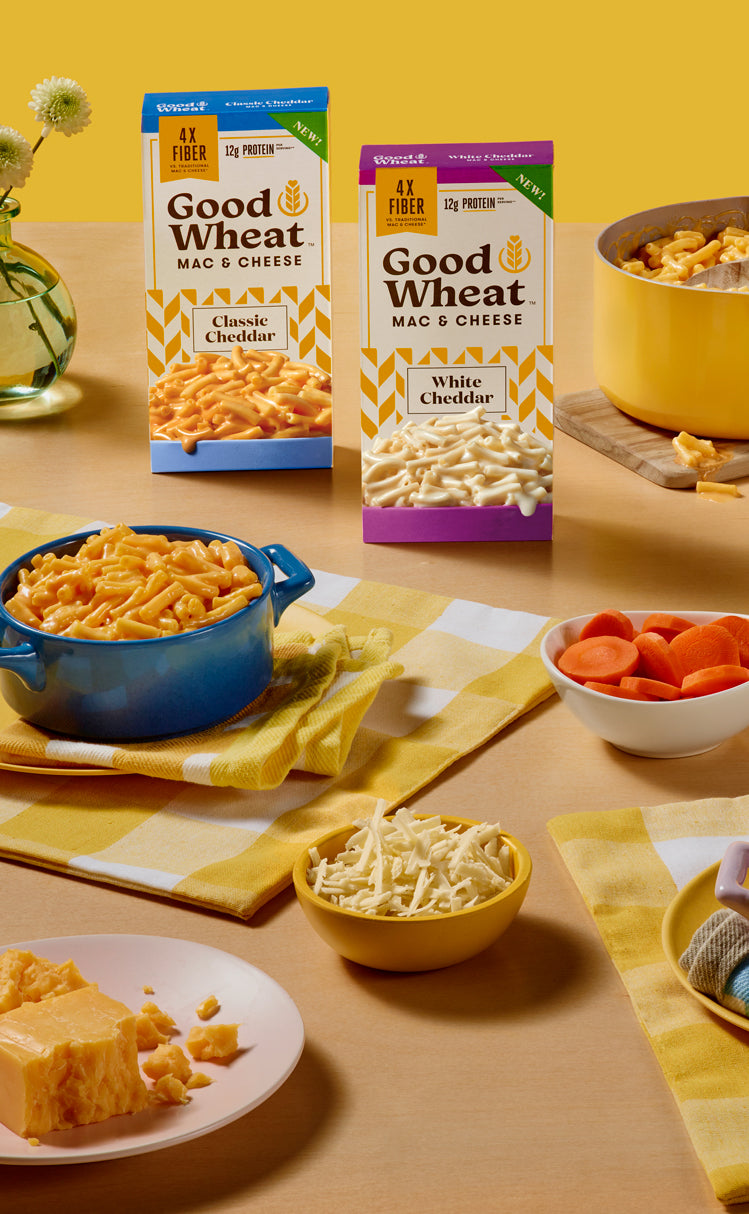This detailed image depicts a visually appealing commercial setup for "Good Wheat Mac and Cheese" products, showcasing both Classic Cheddar and White Cheddar varieties. At the center of the composition, the two boxes prominently feature these flavors: the Classic Cheddar box with blue accents and the White Cheddar box with purple accents, both marked with the “Goodwill” logo.

The display includes colorful kitchen items, enhancing the product's appeal. Positioned on a light tan table, adorned with a yellow and white checkerboard-patterned tablecloth, various dishes are meticulously arranged. On the left side, there's a blue pot with handles brimming with vibrant yellow mac and cheese, while on the right, a larger yellow pot holds more mac and cheese. Additionally, a yellow bowl filled with shredded white cheese is placed at the center bottom, and a white saucer in the lower-left corner displays broken pieces of cheddar cheese.

In the upper-left corner, a glass vase with flowers adds a touch of freshness, contrasting with the culinary setup. Beside the yellow pot on the right, there is a white bowl containing round slices of what appear to be either carrots or sweet potatoes. Completing the display, some chopped fruits, likely papaya, sit in the upper right, alongside a white plate with cheese.

The entire scene is bathed in warm yellow tones, highlighted by a yellow wall in the background, effectively emphasizing the cheesy, inviting nature of the mac and cheese products.